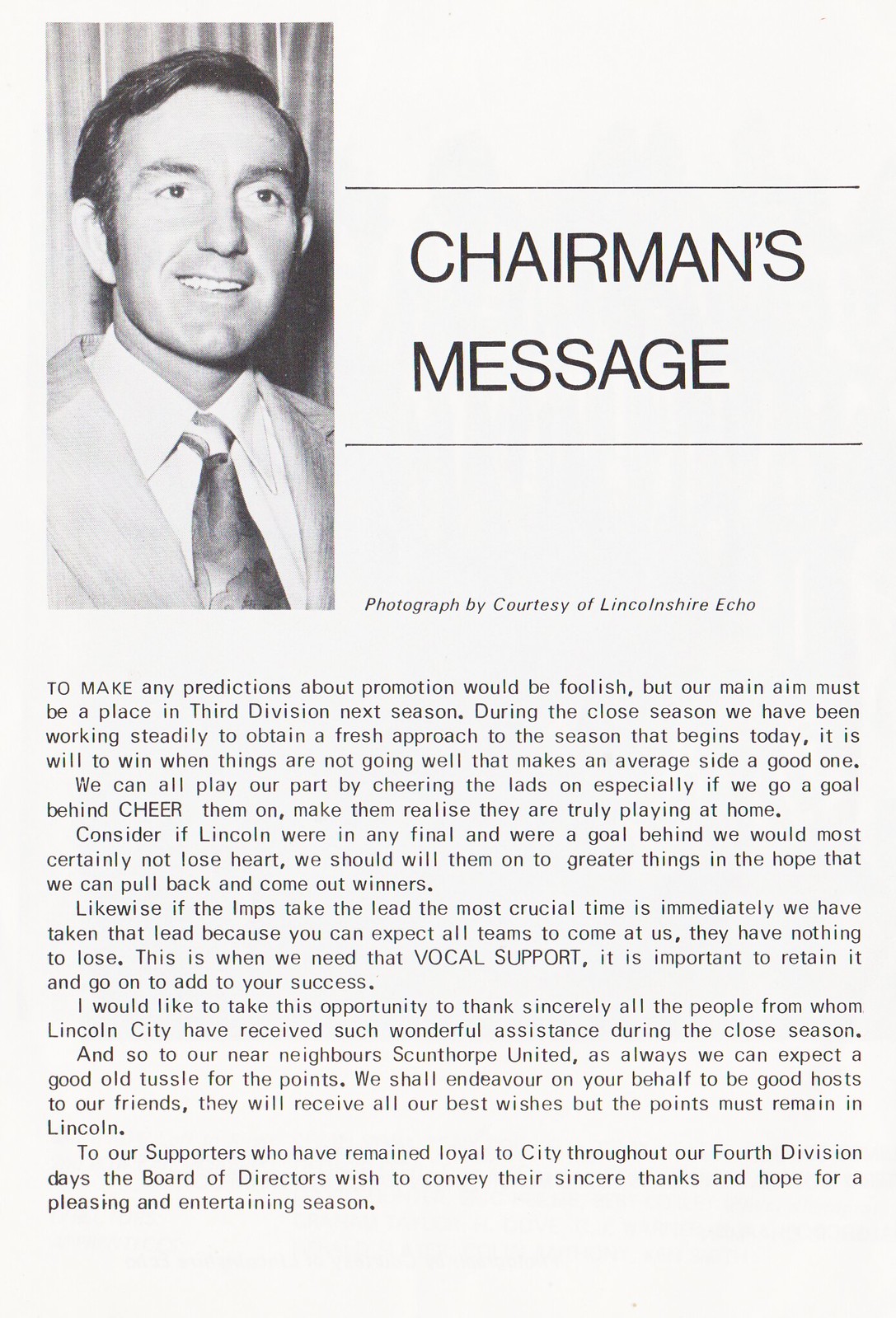This image is an aged off-white or light gray page taken from a publication, likely from the late 1960s or early 1970s, filled with black text headed "Chairman's Message." The page features a black-and-white photograph of a smiling gentleman, a white man with short brown hair, dressed in a suit and tie, which is credited to the Lincolnshire Echo. The chairman’s message discusses the aspirations for the Lincoln City football team, affectionately referred to as ‘the Imps,’ aiming for promotion to the Third Division next season. It highlights the importance of unwavering support from fans, especially during challenging times when the team concedes a goal. Vocal support is deemed crucial both in maintaining a lead and in boosting team morale. Additionally, the chairman sincerely thanks the supporters and all those who assisted Lincoln City during the closed season. He acknowledges the excitement of the season opener and anticipates a tough match against neighbors Scunthorpe United, expressing a hope to retain home points. The message resonates with gratitude for fans’ loyalty throughout the club’s Fourth Division days and optimistically looks forward to an entertaining season.